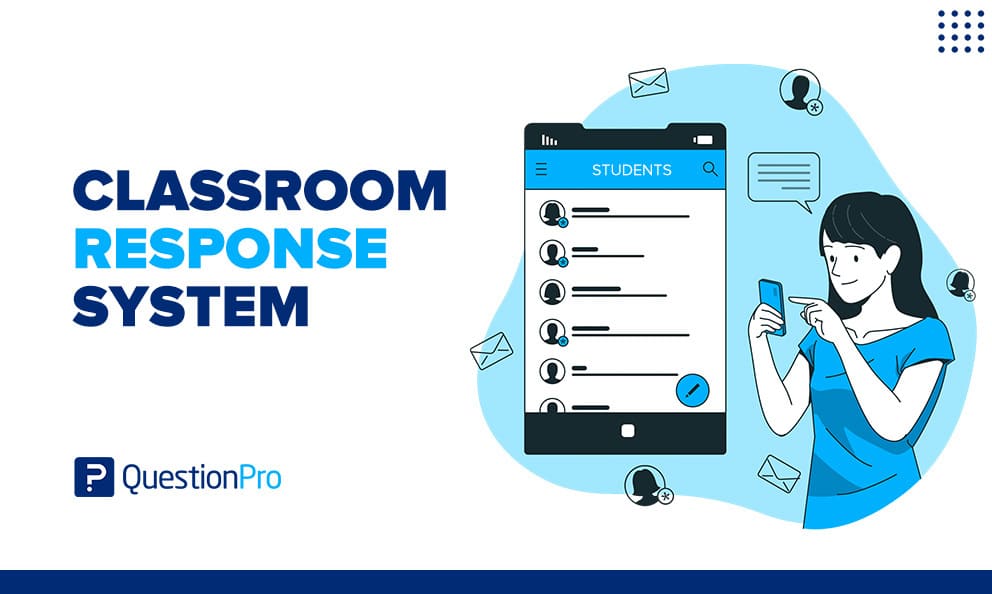The image is a colorful, digital graphic promoting an app called the Classroom Response System, designed for teachers to interact with students via pop quizzes and real-time responses. The central figure, a woman holding a blue phone, appears to be selecting answers, symbolizing student engagement through the app. Surrounding her head are thought bubbles, small envelope icons indicating messages or notifications, and various gendered figures denoting student avatars. 

On the right side, the app interface is depicted, showing a cartoonish screenshot of a student list with pencils and search icons, emphasizing the interactive and organized nature of the system. The graphic prominently displays the title "Classroom Response System" in dark and light blue, with the addition of "Question Pro" at the bottom. The background is predominantly white, complemented by light and dark blue accents, with a solid blue bar running horizontally across the bottom of the image, unifying the overall color scheme.